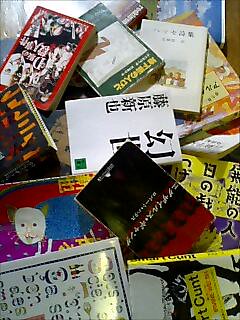The image is a small, low-resolution thumbnail photograph capturing a colorful, haphazard pile of paperback books. These books, appearing in a variety of vibrant hues including white, green, red, orange, blue, purple, and black, are randomly scattered with no apparent order or orientation, as if they were simply tossed onto a table. The scene is viewed from above, showcasing numerous book covers, many featuring Japanese text in dynamic fonts, though a couple display English words — including one partially readable 'C' word. The covers boast diverse illustrations, one notably resembling an animated character similar to Thomas the Tank Engine crossed with a caterpillar. The photograph’s poor lighting and close-up nature emphasize the disarray, making it evident that this is an informal snapshot rather than a professional presentation.